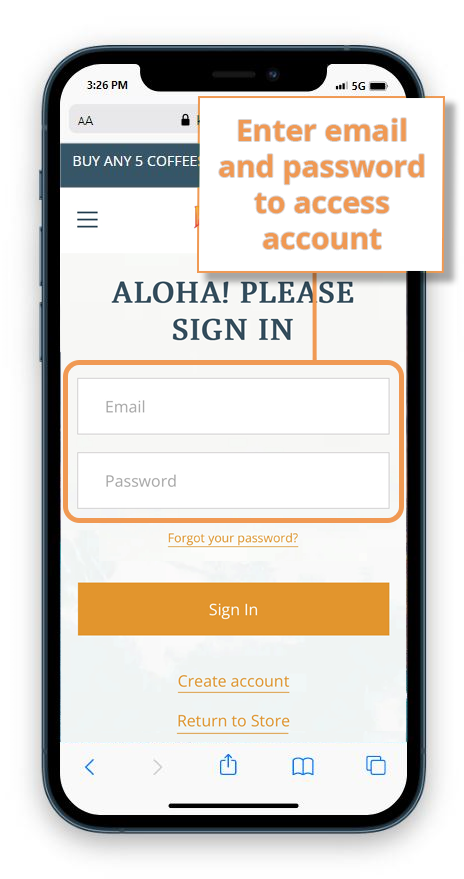The image is a screenshot from the Amazon website, indicating a login page. At the top of the screenshot, several status icons are visible: the battery icon on the far right is fully charged with a black inner color, followed by the "5G" label, and a signal strength icon showing three out of four bars. The top left corner displays the current time as 3:26 PM.

Directly beneath these icons lies the URL bar, though its right side is obstructed by a box. The obstructing box contains the text "Enter email and password to access account," which is colored orange and features a vertical line extending downward around the email and password fields.

Centrally placed on the image is a greeting message stating, "Aloha, please sign in." Below this message are the fields for email and password entry. Further down, there is a prompt reading "Forgot your password?" highlighted in orange with an underline. Another box below it features a "Sign in" button with an orange background and white text.

At the very bottom of the screenshot, two additional links are displayed: "Create an account" and "Return to store."